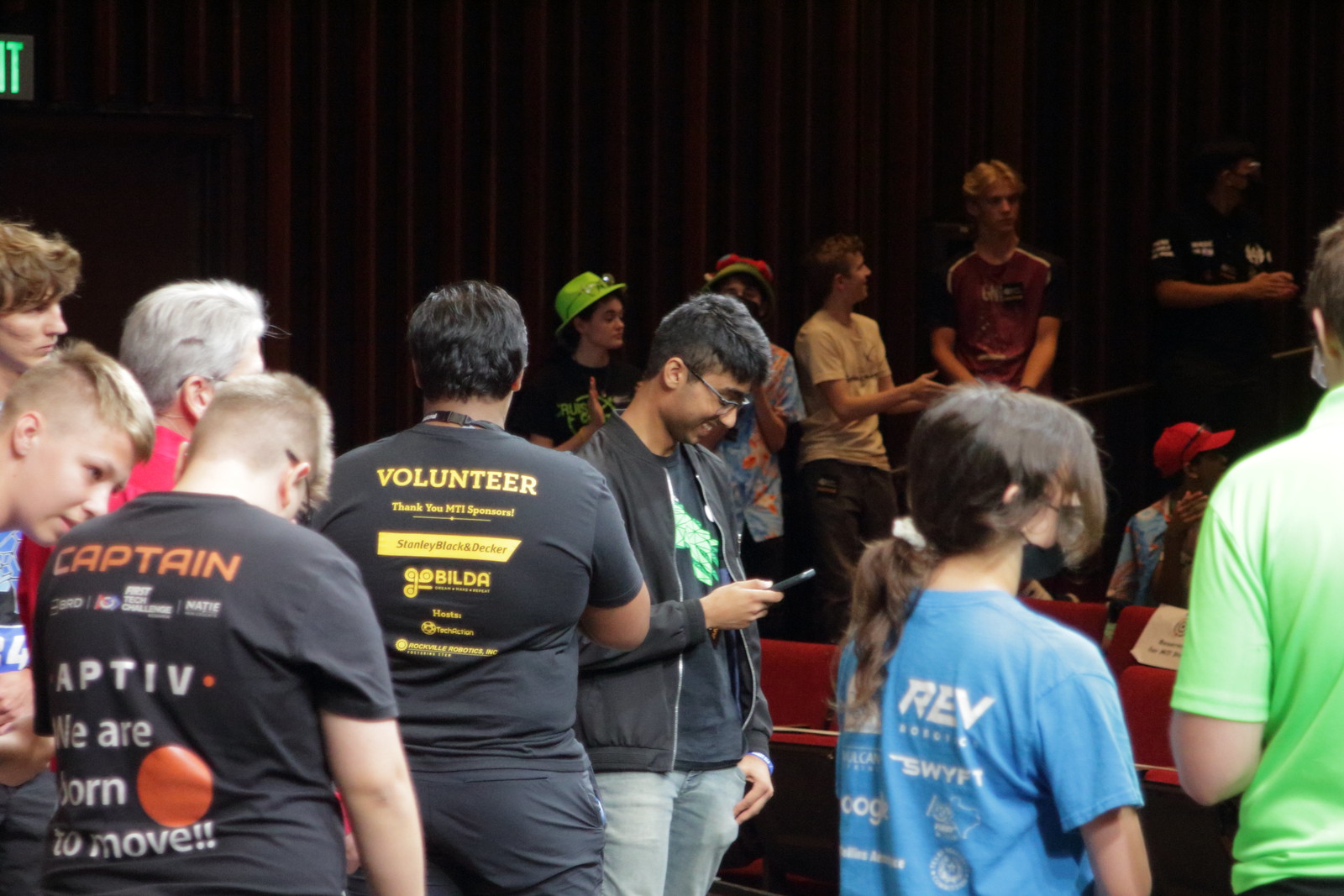The image depicts a bustling scene inside a large room filled with people of various ages, mostly young. Many participants wear shirts of different colors such as blue, lime green, black, red, and tan. The backdrop features dark red curtains, and towards the bottom right, behind the crowd, are theater-style red seats. Central to the image is an individual viewed in side profile, holding a cell phone in their right hand, possibly capturing a moment or texting, while others around them either look at their phones or await something to happen. The text visible on some shirts includes "Volunteers, thank you MTI sponsor, Stanley Black and Decker" and "Captain, we are born to move." The general atmosphere suggests that people are casually gathered, some organized in loose lines, possibly for an event, with a girl in a ponytail and blue shirt noticeable among them.